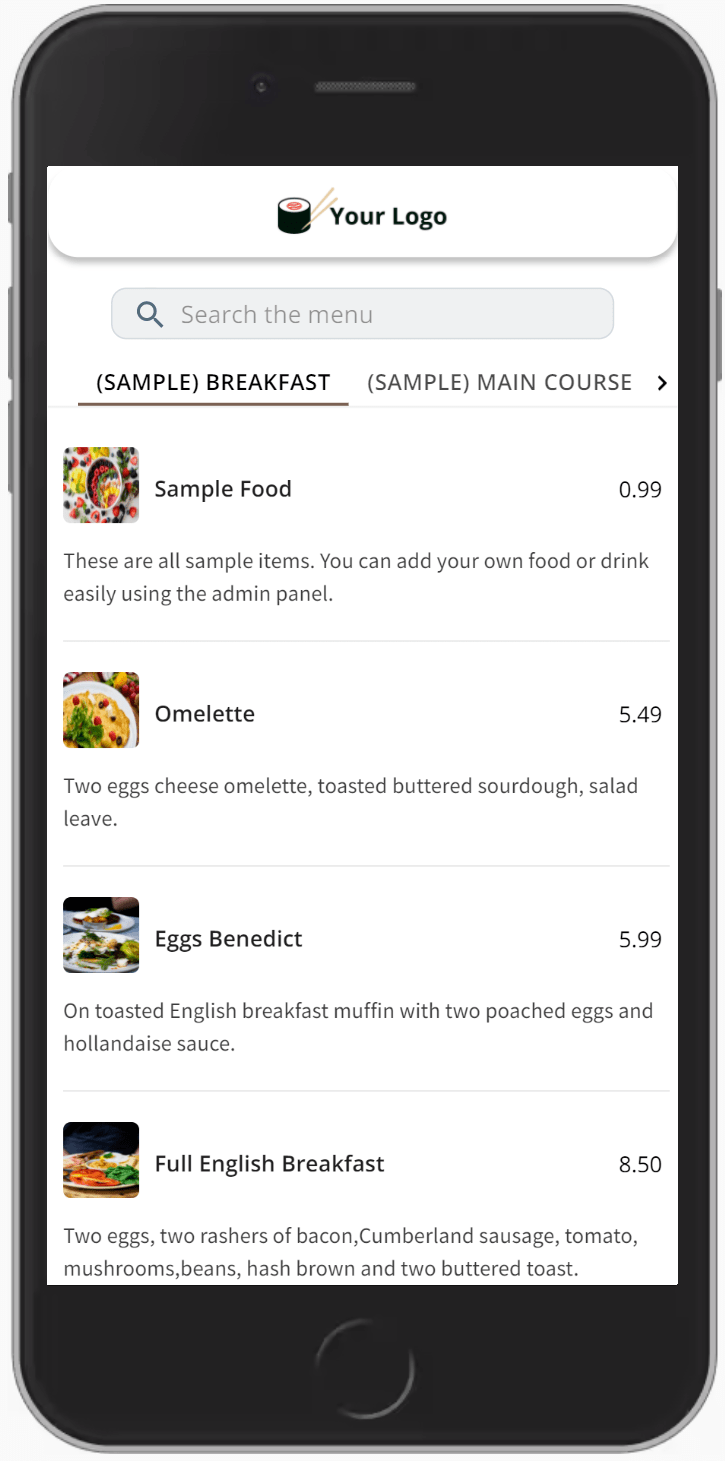The image depicts a mobile website interface showing a food menu that is currently populated with placeholder text. At the top of the page, there is a section labeled "Your Logo," featuring an illustrative logo of sushi with chopsticks. Just below this, a search bar is prominently placed, inviting users to "Search the menu."

The menu is divided into several sections, with the visible sections being "Breakfast" and "Main Course." It appears that there are additional menu sections accessible via horizontal scrolling. The "Breakfast" section lists the following sample items with their respective prices: 

- Sample Food - $0.99
- Omelette - $5.49
- Eggs Benedict - $5.99
- Full English Breakfast - $8.50

Each item is marked as a sample, indicating that administrators can custom-fill the content using an admin panel. Specifically, selecting the "Full English Breakfast" item reveals a detailed list of components included: two eggs, two rashers of bacon, a Cumberland sausage, tomato, mushrooms, beans, hash browns, and two slices of buttered toast.

The design primarily employs brown and black text against a minimalistic, sleek background, enhancing readability and user experience.